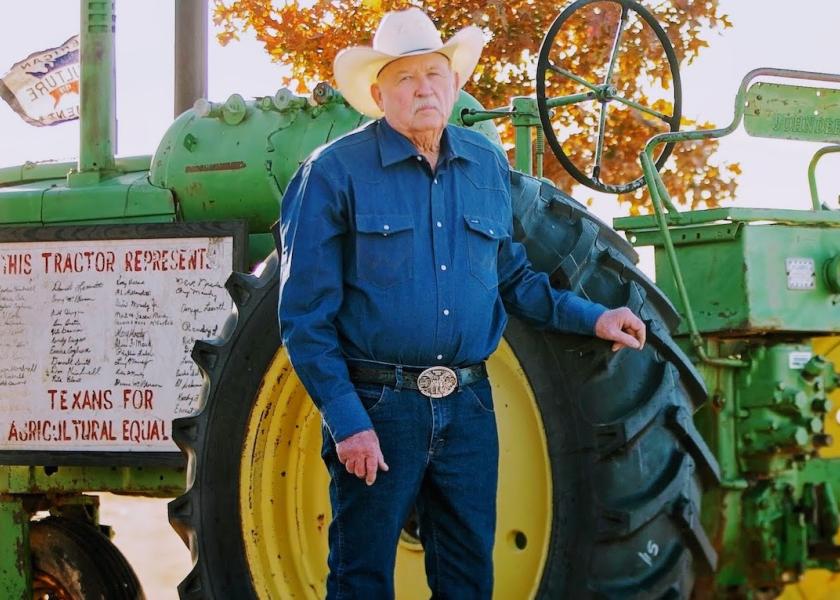In this colorful photograph, an older man stands confidently in front of a large green tractor, bathed in sunlight that illuminates the scene. His attire is typical of a farmer: a light-colored cowboy hat with a black band, a blue buttoned-up collared denim shirt, dark denim jeans, and a black belt with a large, ornate belt buckle. He sports a light-colored handlebar mustache and rests his left hand on the tractor's sizeable black tire, which is mounted on a yellow wheel. The tractor has a noticeable sign on its side with a white background, red text reading "This tractor represents," and "Texans for Agricultural Equality" along with numerous black signatures beneath it. Behind the tractor, a tree with orange or yellow leaves stands out against the clear blue sky, adding a splash of autumn color to the backdrop.